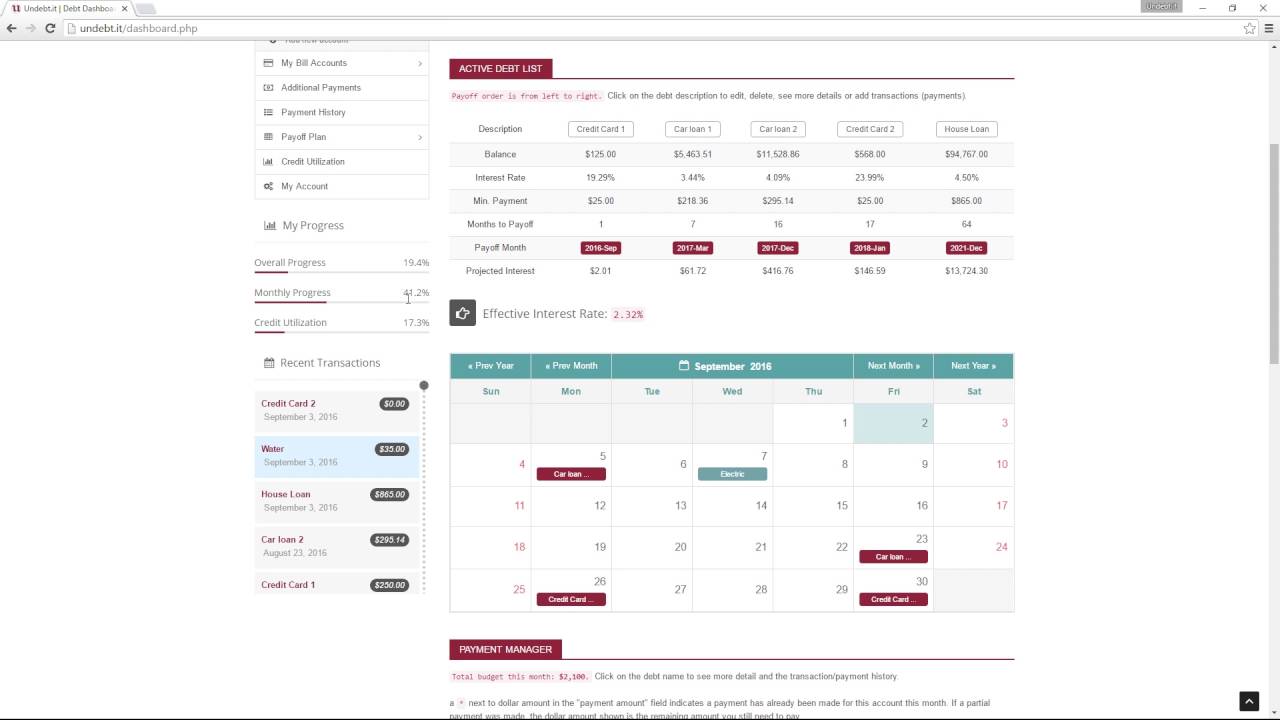The image depicts a screenshot of the Google Chrome browser with a URL box at the top. The webpage shown has a white background with a detailed layout. On the left side, there is a menu containing several clickable options, including some grey buttons. To the right of the menu, there is a prominent red box labeled "active." Adjacent to the red box is a line with text beneath it. Below this section, there is a graphical representation, with various inputs aligned on the left. At the top, there are five distinct boxes with numbers underneath them. Further down the page, within the second column from the bottom, there are red rectangular-shaped boxes with text inside them. Lastly, there is a calendar display at the bottom of the image, featuring a teal header and several days marked with red boxes.